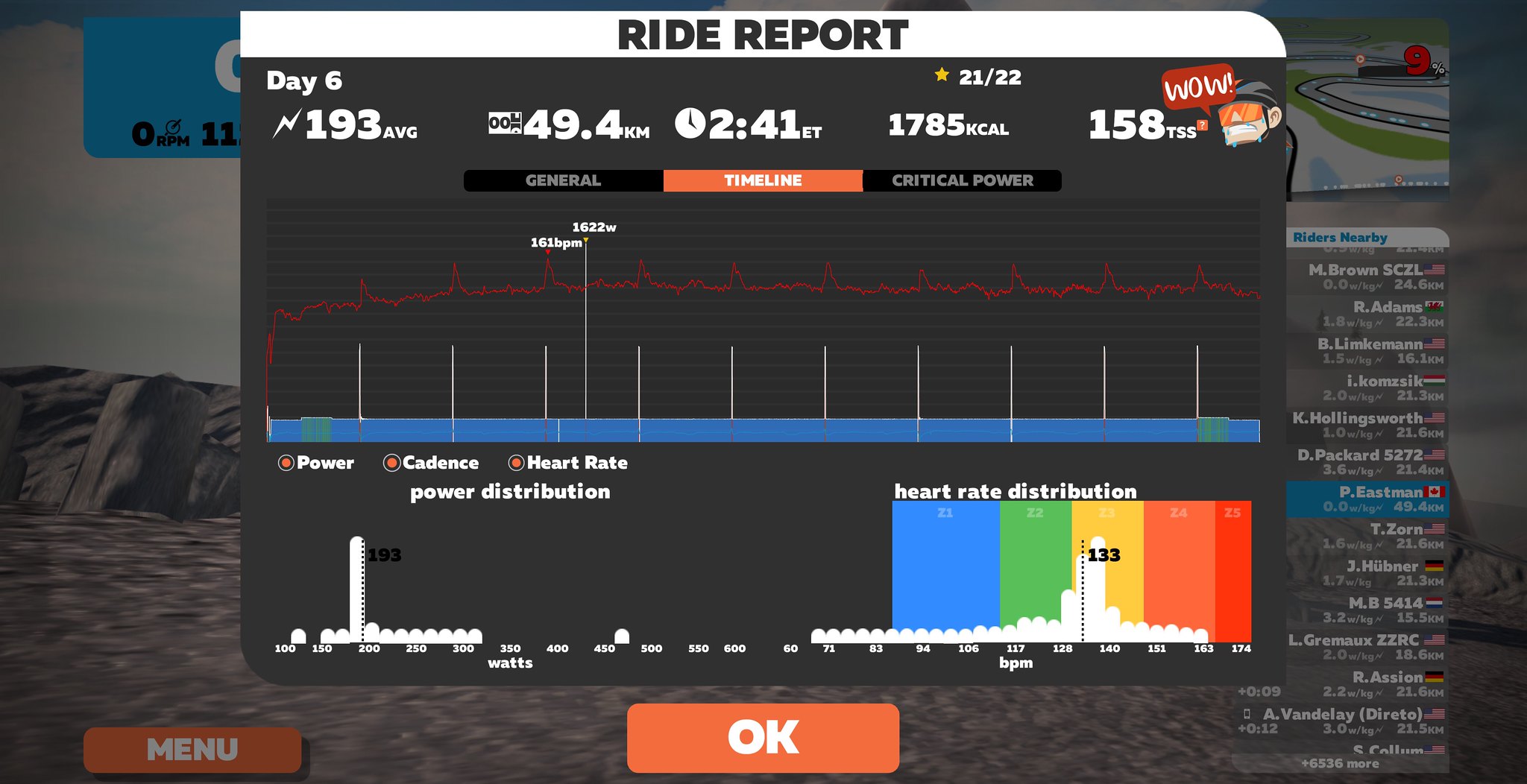The image displays a detailed ride report from a computer app designed for eBikes, tracking various metrics while riding. At the top, the report is labeled "Ride Report" with a standout "WOW" above, highlighting an impressive performance. Key statistics for day 6 are prominently shown, including an average of 193 with a lightning bolt icon, 49.4 kilometers covered, and the time recorded at 2:41 Eastern Standard Time. Other critical data points include 1,785 kcal burned and a TSS (Training Stress Score) of 158, acknowledged by a yellow star next to "21-22".

A chart is segmented into three categories: General, Timeline, and Critical Power. Data visualization includes a red frequency indicating a heart rate of 161 BPM and a white indicator showing a peak power of 1,622 W. Below the chart, various metrics such as power, cadence, heart rate, power distribution, and heart rate distribution are outlined.

In the bottom right corner, multiple colors (blue, green, yellow, orange, and red) likely represent different performance zones or thresholds. The interface features buttons labeled "Menu" and "OK" at the bottom, enhancing user interaction. This comprehensive app not only tracks extensive ride data but also motivates users by displaying flags of other nearby riders, suggesting its utility in competitive eBike racing scenarios.